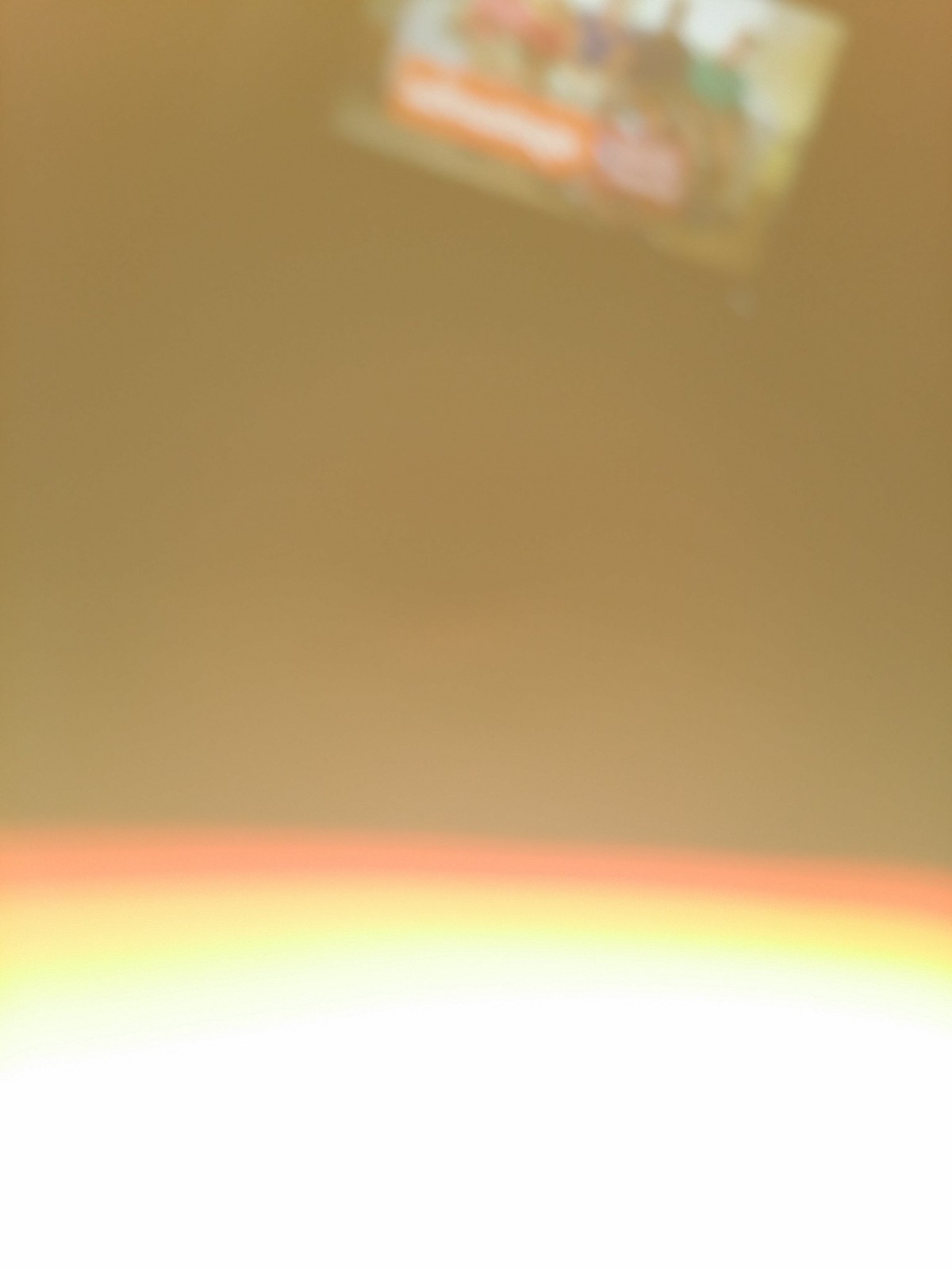The image primarily features a large expanse of light brown, solid color without any distinct texture. Dominating the lower portion of the image are a series of parallel bands that arch slightly from left to right. From top to bottom, these bands include a strip of white, followed by a gradient of light yellow transitioning into a deeper yellow, and finally a band of orange. At the very top of the image, a slightly out-of-focus rectangular object extends off the upper left corner of the frame. This object appears to feature a picture, possibly depicting people in a line. An orange rectangle within this object contains a white area, likely meant for text, though it appears as an indistinct orange and white blob.